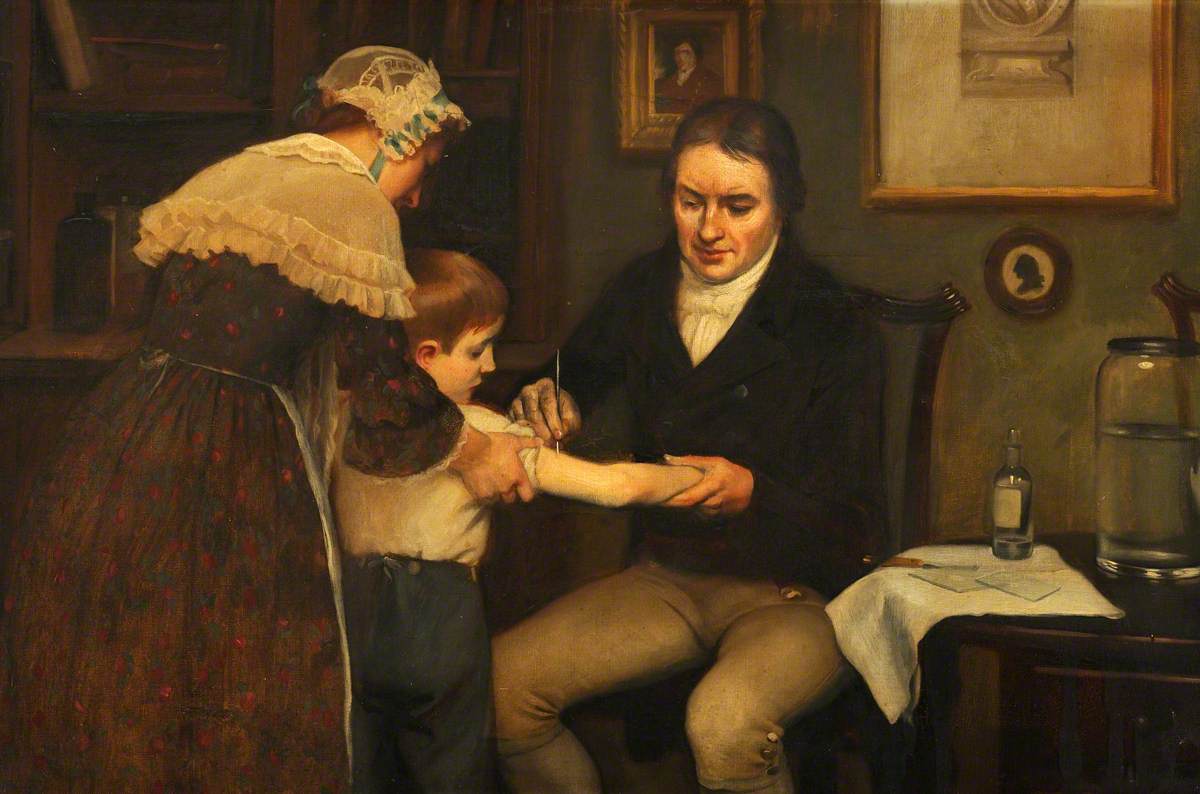This painting, seemingly set in post-colonial America, portrays a tender yet serious scene from a past era. In the center, a woman dressed in traditional attire, adorned with intricate lace and a head wrap, gently holds the arms of a child, who appears to be around eight or nine years old. The child stands between the woman and a man who is seated. The man, engrossed in his task, carefully holds one of the child's arms as he applies a pen or possibly administers medicine. The scene suggests a moment of teaching or a medical procedure.

The background features period-appropriate decor, including framed portraits that enhance the historical ambiance of the room. On a nearby desk, various objects—a jar of water, a small bottle of elixir, and an assortment of tools and sheets—are meticulously arranged, hinting at the man's trade or practice. The overall composition conveys a meticulous, almost ritualistic atmosphere, reflecting the customs and challenges of the time.